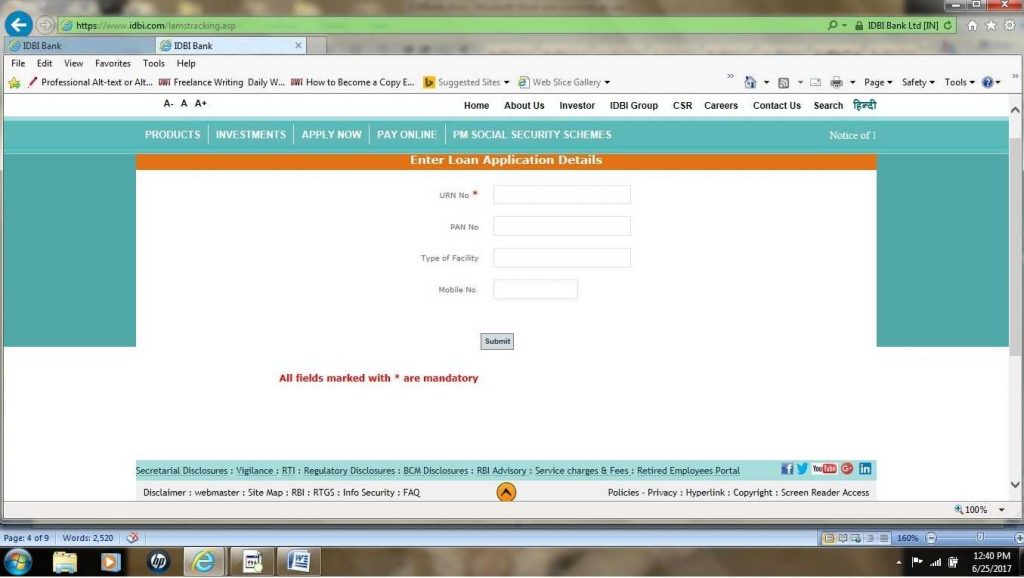The image features a partially maximized web browser on a computer screen, displaying various desktop elements and a banking website.

In the background, the Windows taskbar is visible at the bottom of the screen. Iconography includes the Windows logo, a folder icon, a music media player icon, and a blue-and-white circle, likely representing an HP application. The system clock indicates the time is 12:40 PM, and the date reads June 25, 2017. A white charger symbol suggests the laptop is plugged in and nearly fully charged.

The web browser—an older version of Internet Explorer (indicated by the two open tabs)—is in focus. The active tabs are labeled "IDBI Bank." Below the address bar, there are familiar menu options like File, Edit, View, Favorites, Tools, and Help.

The website itself is for IDBI Bank and features a navigation bar with links labeled Home, About Us, Investor, IDBI Group, CSR, Careers, Contact Us, and Search on a black background. Below this, a teal-colored section with white text offers additional links, such as Products, Investments, Apply Now, Pay Online, and possibly 'PM Social Security Schemes.'

Further down, an orange banner with white text prompts users to "Enter loan application details." The form underneath includes various input fields labeled "You are N and O," "PAN and O," "Type of facility," and "Mobile and O," followed by a gray "Submit" button.